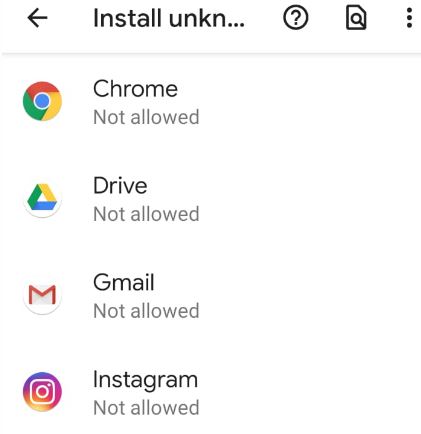In this image, we have a screenshot depicting a user interface. At the top of the interface, there is a header that reads "Install," though the word "Install" appears partially cut off with an ellipsis ("...") suggesting the presence of more text, likely the word "Unknown" or something similar. To the left of this header is a back button, and on the right side are three icons: a circle with a question mark inside, a search button, and a menu represented by three vertical dots.

Below this header section, there are four listed applications, each with its respective name and icon. The applications, from top to bottom, are Chrome, Drive, Gmail, and Instagram. Each app icon is displayed within a circular symbol to the left of its name. Beneath the name of each application, there is text in gray that reads "Not allowed," indicating some form of restriction for these apps.

The right side of the screen displays a plain white background without any scroll bar or mouse pointer, suggesting that this is a static list without immediate interaction tools or additional navigation elements.